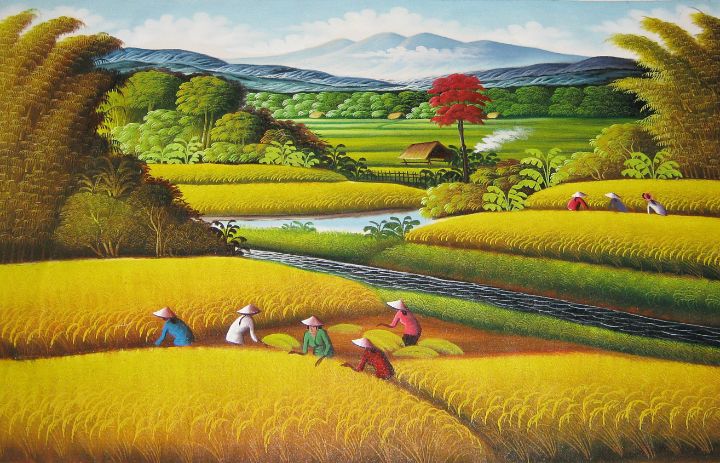This is a detailed painting depicting a rural scene with a group of laborers working in expansive cornfields. The foreground prominently features workers kneeling and wearing distinctive pink lampshade-type hats. These laborers are dressed in various colored shirts, including red, white, and gray. The fields they tend are vibrant yellow and towering, with three additional workers visible in the right section. The background adds depth with a lush green environment, a prominent red tree that stands out among the greenery, and distant mountains with snow-capped peaks under a blue sky with scattered clouds. A calming river runs through the center of the scene, dividing the cornfields. Additionally, there's a triangle-shaped building, likely a barn, situated in the background, and a subtle fence line provides further context to the rural setting. The rich color palette includes reds, blues, greens, light greens, light yellows, browns, tans, and whites, capturing the essence of a serene, sunny day.